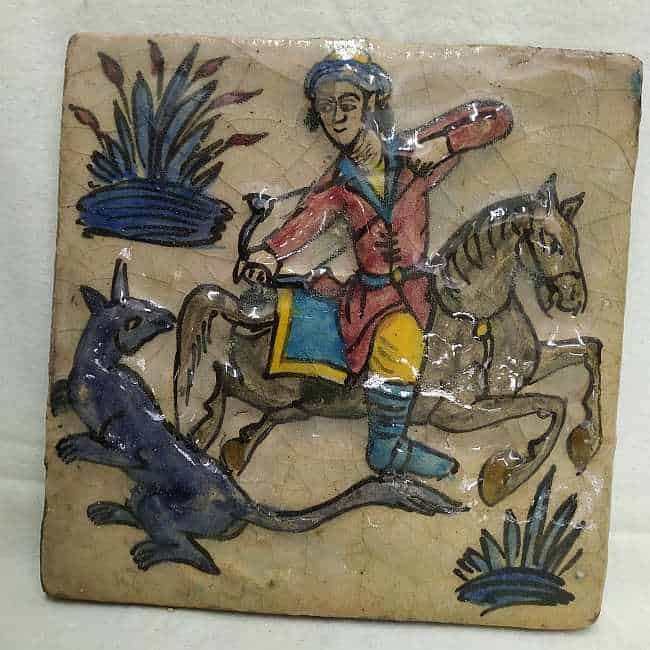The image depicts a detailed ceramic tile artwork set against a white backdrop, showcasing a vividly colored medieval scene. Central to the artwork is a young archer, adorned in a red coat with blue lapels, yellow pants, and blue riding boots, mounted on a galloping brown horse. The archer, wearing a blue and yellow hat, twists around in his saddle, aiming his drawn bow and arrow at a mythical creature on the tile's left side. The creature, resembling an amalgamation of a dog and a fox with a single horn, is colored blue. The tile itself has visible grazing lines and appears either vintage or designed to look aged, with a few cracks adding to its character. Additionally, two blue potted plants with fronds are situated on the top right and bottom right of the tile, enhancing the scene's intricate medieval design.